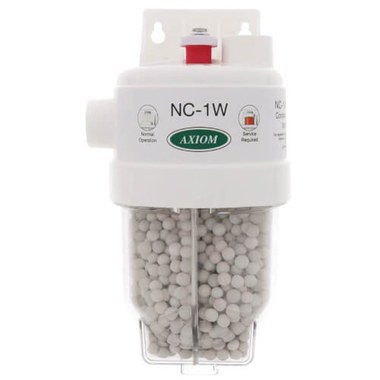The image depicts a vertically positioned plastic device, possibly an industrial filter or water filtration component, filled with small gray pebble-like beads. The device, which features a white cap and additional white parts protruding from its plastic structure, prominently displays the text "NC-1W" and bears the Axiom logo in a green oval. Accompanying the text are two small diagrams on either side; one completely white, and the other red with a white top, corresponding to the device's placement in the red and white-topped section. The overall color scheme includes white, red, gray, green, and black, set against what appears to be a white background, suggesting that the photo was likely taken for retail or resale purposes. Some smaller text is also present but remains illegible.